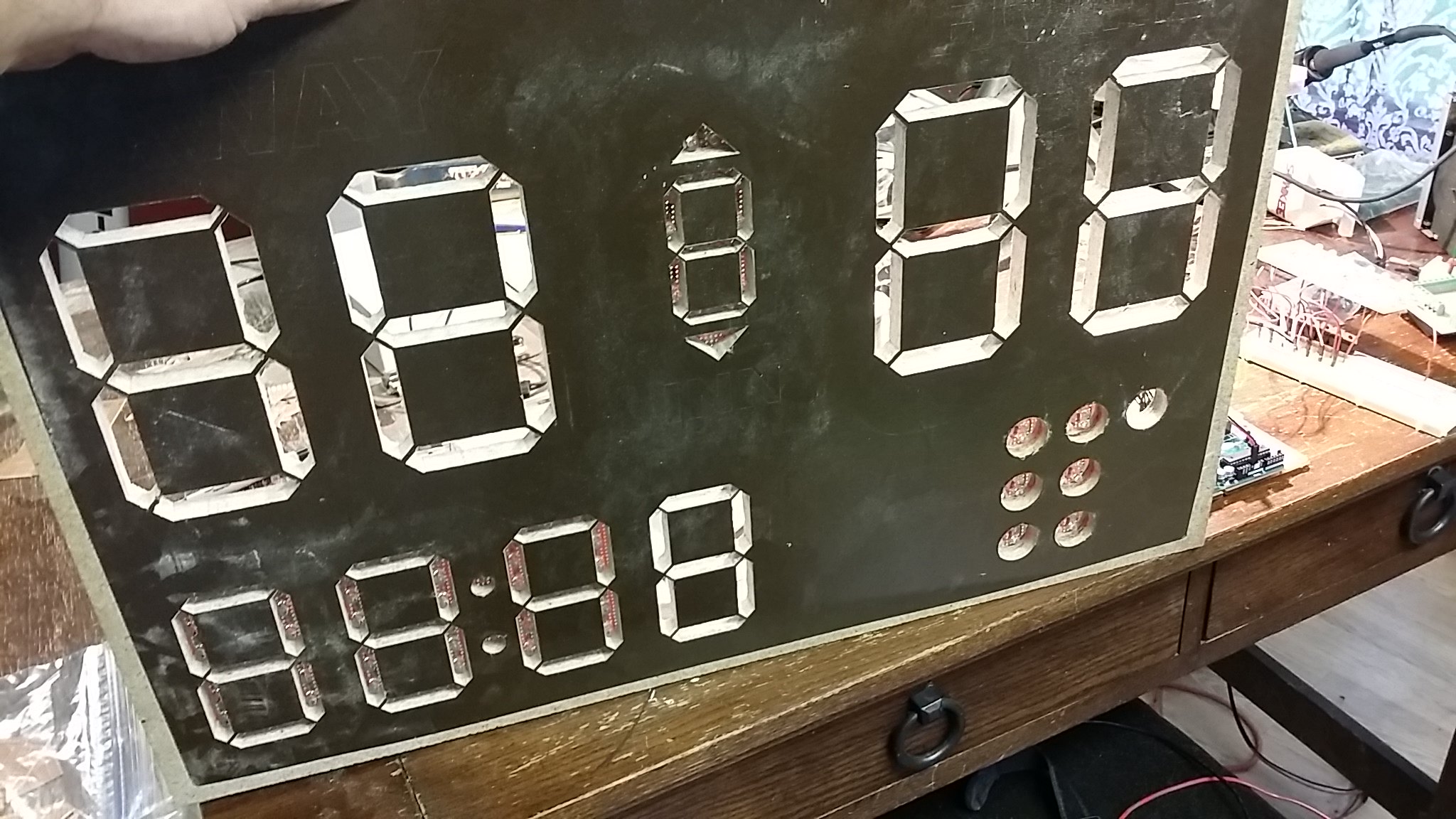The image features an unlit scoreboard device set atop a brown wooden table. The scoreboard's background appears black, reminiscent of a chalkboard. Displayed prominently in the center are numbers formed by eight digits, creating an "88:88" display. Surrounding the central numbers are seven circles, each containing distinct images or icons. Additionally, various small, unrelated items are scattered in the background on either side of the scoreboard. The overall setting suggests a mix of electronic and manual elements, all situated against a dark, chalkboard-like backdrop.